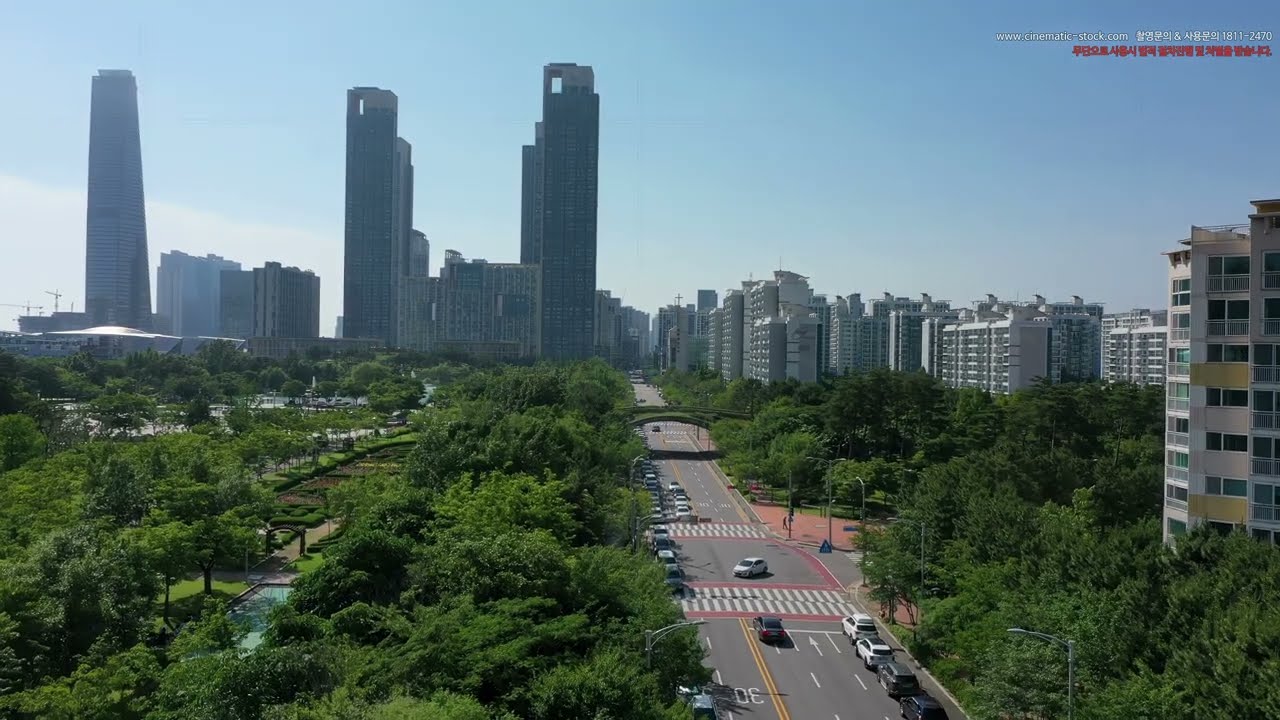This image captures a bustling downtown cityscape with a distinctly urban yet green aesthetic. Dominating the left side of the skyline are three towering skyscrapers, each rising to approximately 40-50 stories and clad in shades of gray and blue. These skyscrapers overshadow several smaller buildings which range between 10-20 stories. An aerial view reveals an expansive avenue, a four to five-lane highway that cuts through the heart of the city, flanked by lush green spaces and a park. The road, dotted with parked cars and lightly trafficked, is crossed by an arched bridge and lined with trees, adding to the city's well-planned design. Two white walkways, bordered in red, are visible on the avenue and are populated with pedestrians strolling along the sidewalks. A small fountain punctuates the greenery, adding a touch of tranquility. The sun shines brightly, casting a light blue hue across the sky. In the upper right corner of the photograph, there is a watermark stating "www.cinematic-stock.com" followed by characters likely in a foreign language, possibly Korean.